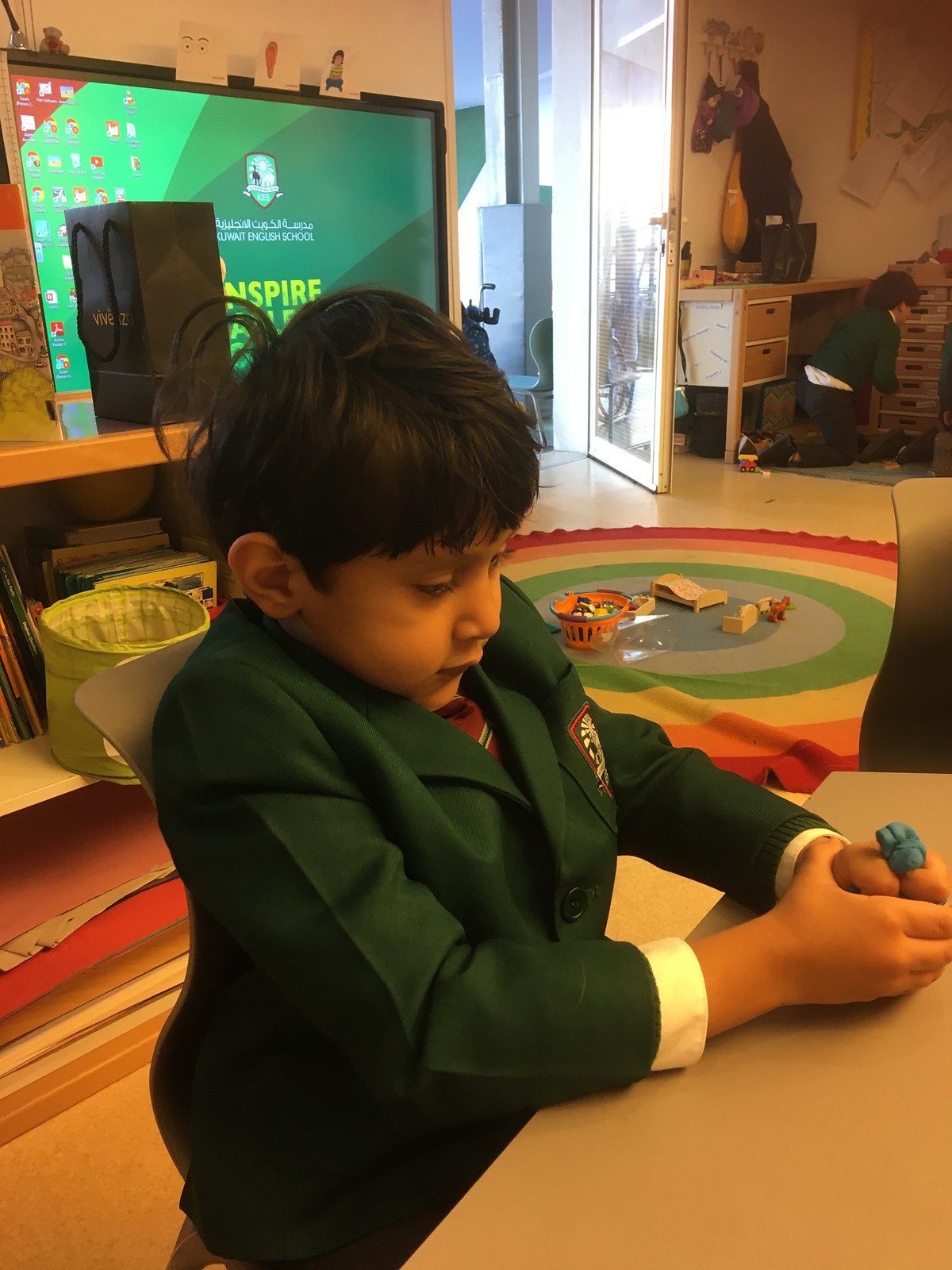In the image, a young boy, likely between 8 to 10 years old, is standing in an indoor setting that appears to be a classroom or playroom. He is dressed in a dark green jacket that resembles a suit, complete with a red tie featuring white and blue stripes. His white shirt under the jacket complements his semi-formal attire. On the right breast pocket of his jacket is a partially visible emblem with a red outline, resembling the top part of a pharaoh's head. The boy's hair is slightly messy, suggesting he might be coming from a recent event.

He is engaged in a playful activity at a table, handling a piece of Play-Doh with his left hand forming a fist around it and his right hand cupping it. Behind him, a television screen displays the words "Kuwait English School Inspire" with some additional text that is cut off, indicating a connection to an educational environment. Adjacent to the TV screen, on its right, is a bookshelf and a table with a computer monitor showing a desktop, further indicating the setting might be a classroom.

To the right of the boy, a circular rainbow-colored rug is visible, adorned with various children's toys. There is also a green bucket and a small black box, potentially a piece of electronic equipment, placed above the bucket. In the background, there is an open door letting in natural daylight, providing a glimpse of another room. The photo is a vertical rectangular shot, with the boy positioned from his hips up to the top of his head, facing to the right, while the television occupies the top left corner of the image.